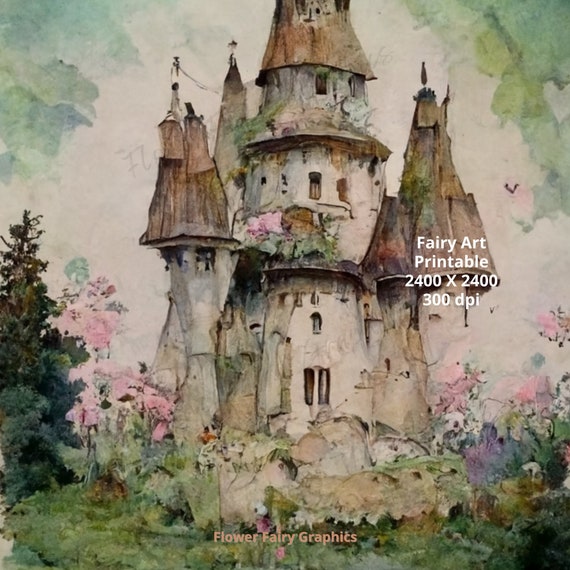This illustrated image depicts a whimsical fairy-tale castle, reminiscent of classic storybook scenes. The castle, crafted from gray slate stone, features multiple turrets topped with rust-brown roofs. Small windows are scattered across its layered façade. The base of the castle is adorned with vibrant pink and purple flowers that intertwine with lush greenery. A tall, dark green evergreen tree stands to the left, while rocks and diverse foliage fill the foreground. The sky above is a mystical blend of blues, greens, and whites, adding to the ethereal atmosphere. The image appears to be rendered in watercolor, enhancing its dreamy quality. Words are visible on the image: "fairy art printable 2400 by 2400 300 DPI" in white text and "flower fairy graphics" at the bottom center. The castle's door is indistinct, contributing to the overall whimsical and slightly blurred aesthetic that invites imagination.